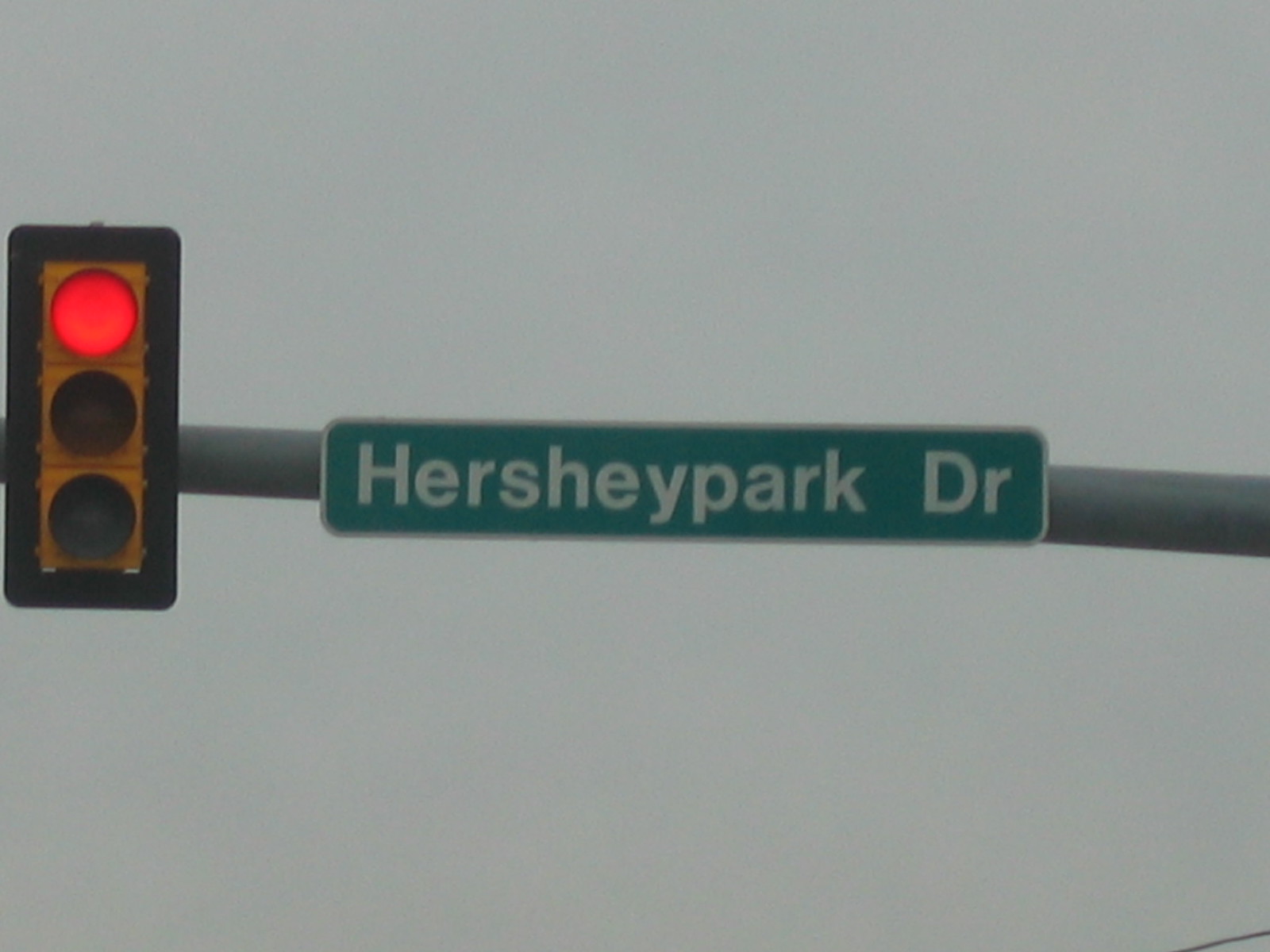This photograph captures a scene focusing on a horizontally oriented, gray metal pole. Mounted on the left side of the pole is a stoplight featuring a black rim and a yellow center section that houses three light indicators. The top light is illuminated in red, signaling for traffic to stop, while the bottom two lights remain unlit and black. Adjacent to the stoplight hangs a green street sign, bordered in white and inscribed with the text "Hershey Park Drive" in bold white letters. The setting is an overcast day, with the sky and background enveloped in shades of gray, emphasizing the weather conditions and adding a somber mood to the image.